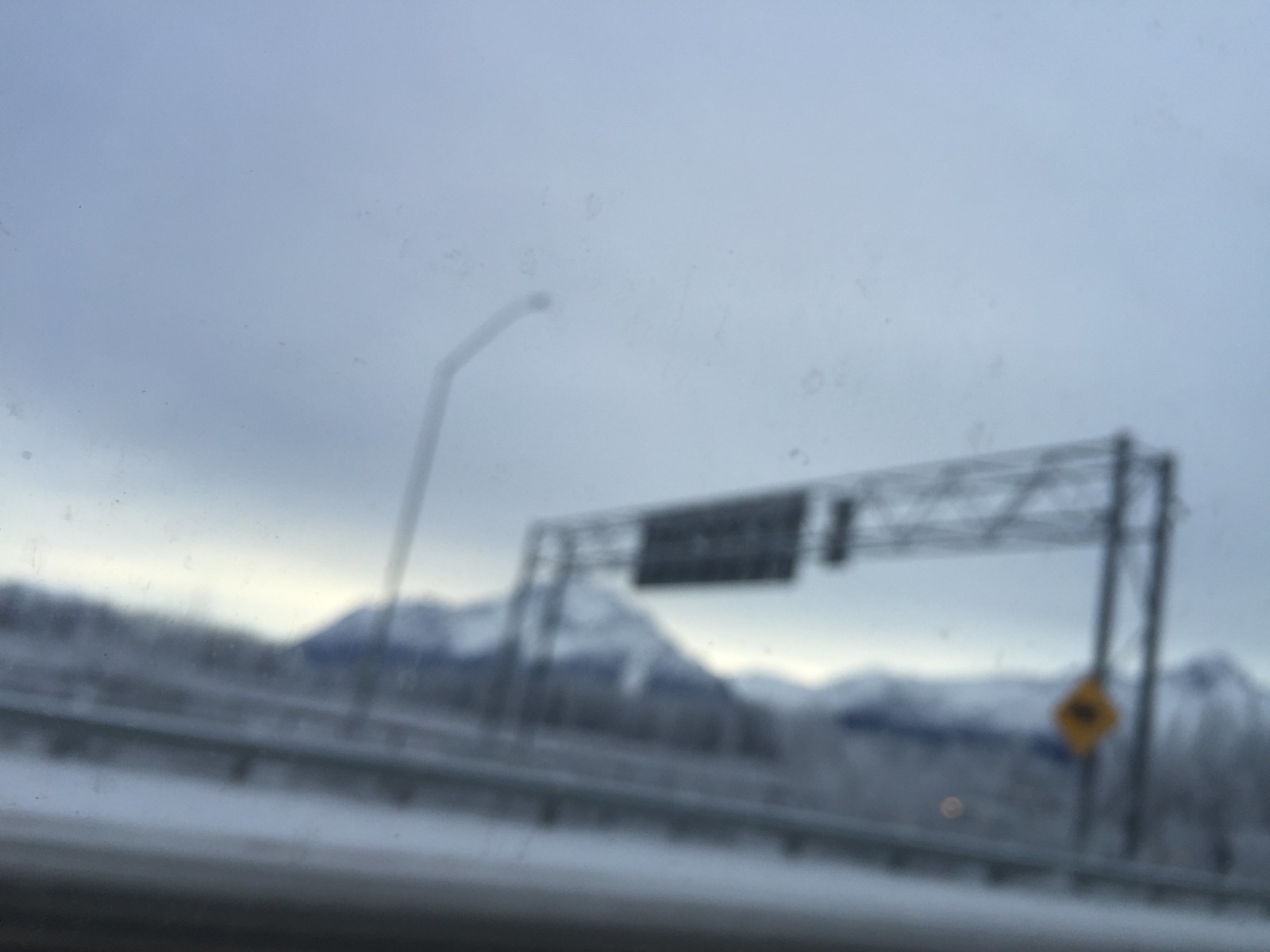A blurry photograph captures a scenic mountainous landscape from a roadside perspective. The upper portion of the image showcases a gray, overcast skyline, adding a dramatic tone to the scene. The bottom half reveals a snow-blanketed black road, bordered by metal guardrails that run across the image. A distinctive yellow caution sign with a black symbol in its center, shaped like a diamond, is prominently attached to an overhead roadway structure. Adjacent to the sign, slightly to the left, stands a solitary streetlight. In the background, snow-capped mountains rise majestically, creating a picturesque but somewhat obscured backdrop due to the blurriness of the photograph.